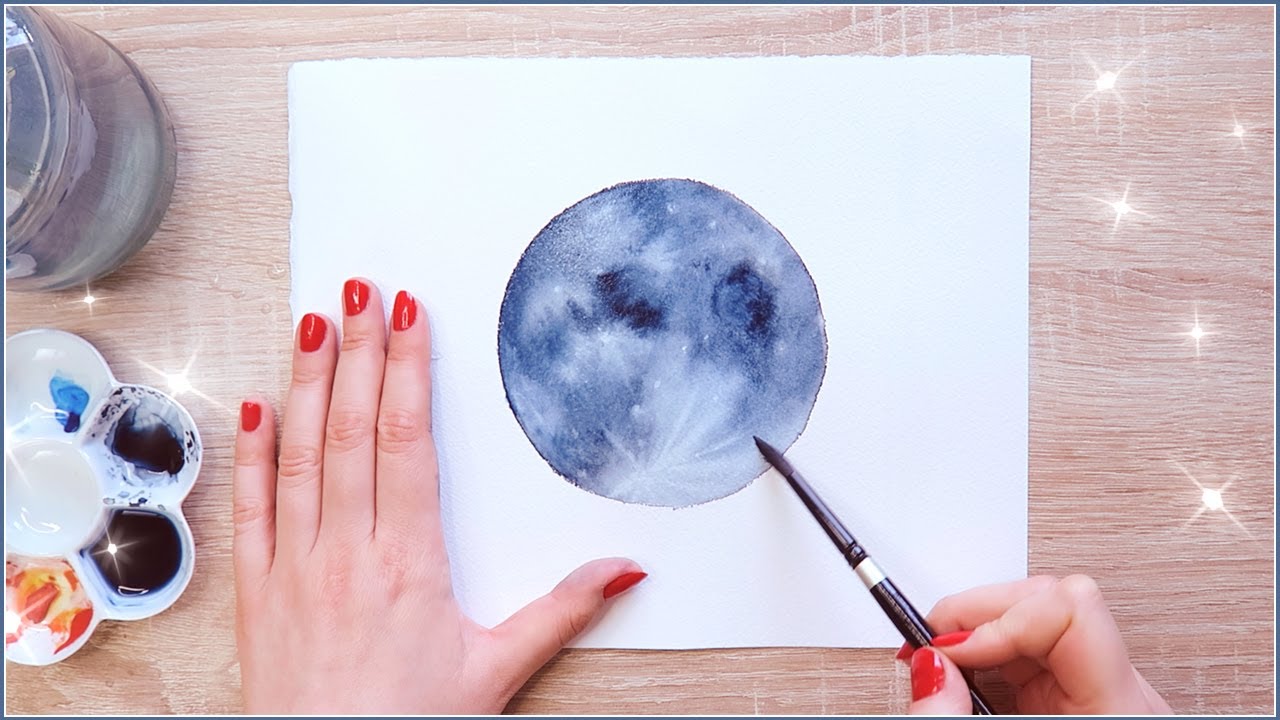In this close-up photographic image, a woman with bright red fingernails is meticulously painting a blue moon on a horizontal white piece of paper. She uses a black brush with a silver band held in her right hand to apply various shades of blue and white to create a vibrant, almost marble-like effect. Her left hand steadies the paper. To her left, there's a small dish divided into compartments containing blue, black, and red paints, accompanied by a jar of water. On the bottom right edge of the paper, three stars have been digitally added, enhancing the celestial theme. The scene is set against a wooden table, providing a warm and natural backdrop to her artistic endeavor.